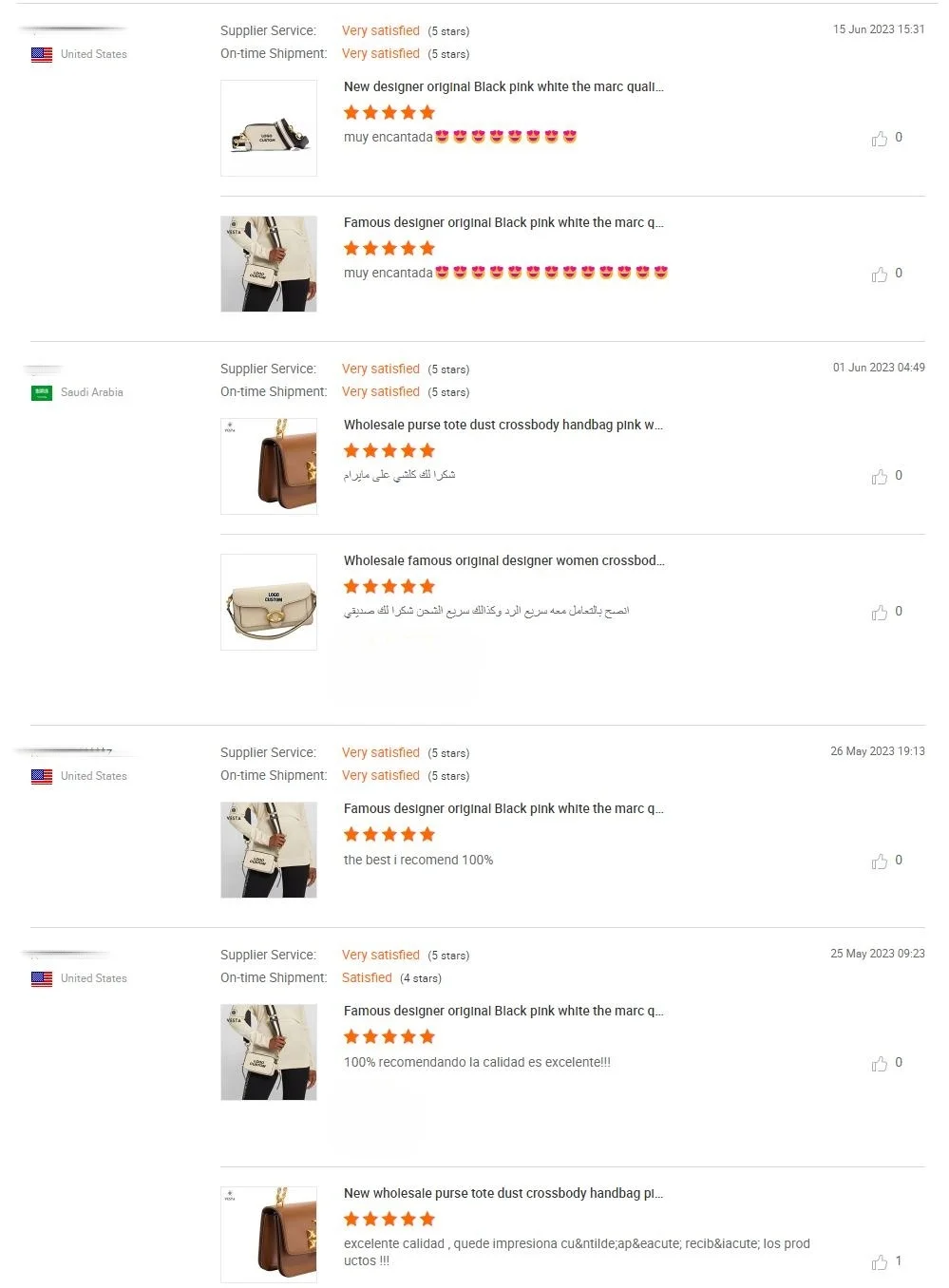The page features a variety of handbags displayed on a clean, white background, primarily using black text with occasional red highlights for emphasis. Each handbag has its own image, with some showcasing a woman modeling the bag. Star ratings are prominently displayed, providing an easy way to gauge customer satisfaction through reviews.

The reviews are visually engaging, with some featuring emojis such as heart-eyed faces to indicate high levels of approval. Each review includes a date, alongside thumbs-up icons with numbers indicating how many users found the review helpful. The national flags of reviewers' countries, predominantly from the United States, but also including Saudi Arabia, are shown next to their comments.

Handbag colors range from brown to cream, with some text in different languages, reflecting a diverse customer base. Additionally, the page offers insights into the shipping timeliness and the quality of the supplier’s service, making it a comprehensive shopping experience.